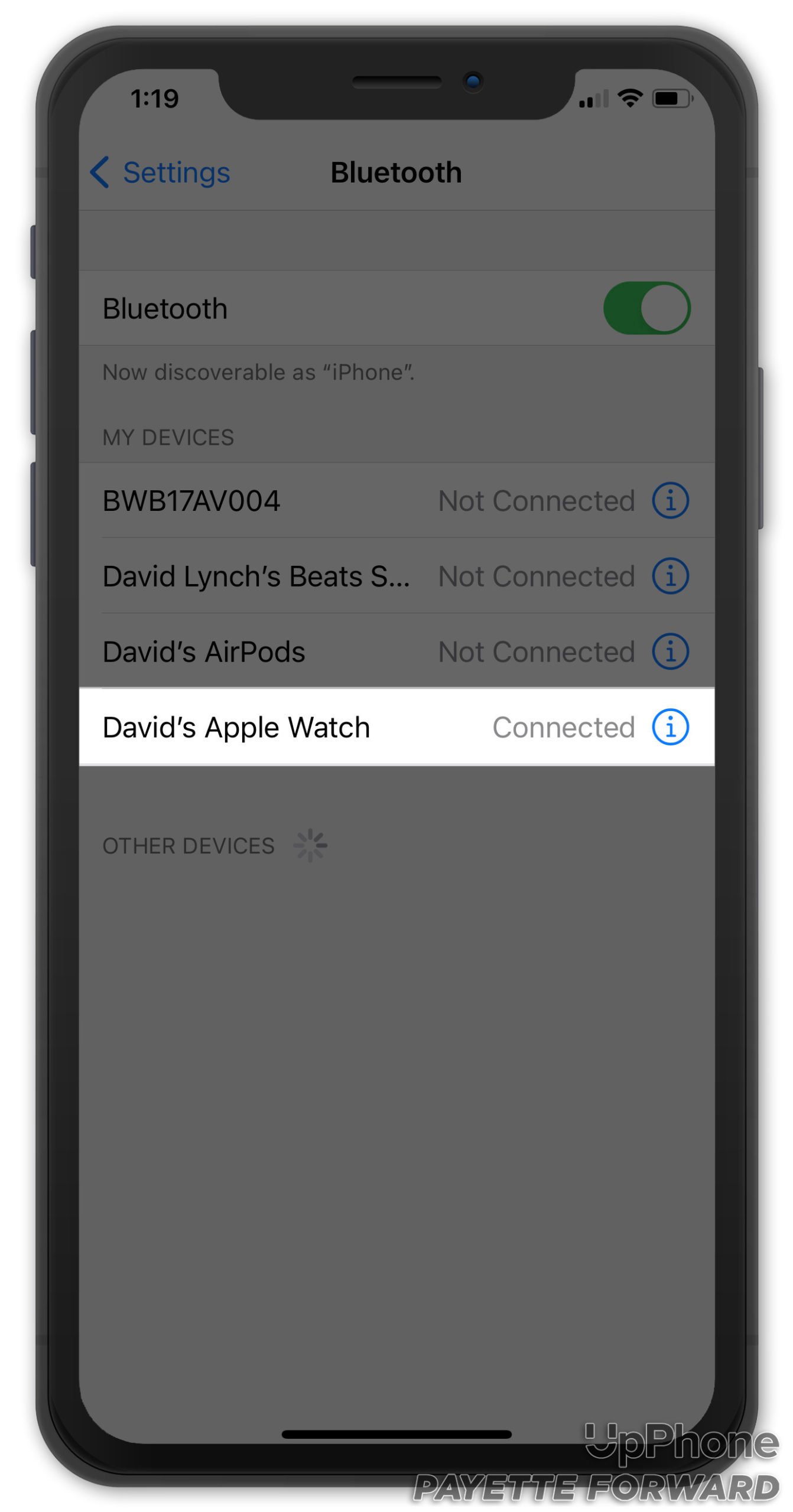This image captures a close-up view of a smartphone screen displaying the Settings tab. The timestamp on the screen reads 1:19. At the top, icons for Wi-Fi and battery are visible. 

At the very top of the screen, in blue text, there is a left-facing arrow labeled "Settings." Centrally positioned in black text is the word "Bluetooth," indicating the sub menu being shown. The Bluetooth toggle switch is positioned to the right and is green, indicating that Bluetooth is turned on.

Directly below the toggle, there is a notification stating, "Now discoverable as 'iPhone'." Below this, the section titled "My Devices" begins, listing several Bluetooth devices with their connectivity statuses. The first listed device, "BWB17AV004," is marked as "Not Connected." Following this, "David Lentz's Beats S" and "David's AirPods" are also shown as "Not Connected." The only device highlighted and labeled "Connected" is "David's Apple Watch." Each listed device has an informational (info) icon next to it, depicted as a sky blue circle with an "i" in the center.

Further down, another section named "Other Devices" appears, although individual devices are not listed within the provided section of the screenshot. 

At the very bottom of the screen, the words "UpPhone" and "Payette Forward" are visible. "UpPhone" is rendered as one word, while "Payette" is spelled as P-A-Y-E-T-T-E, followed by "Forward."